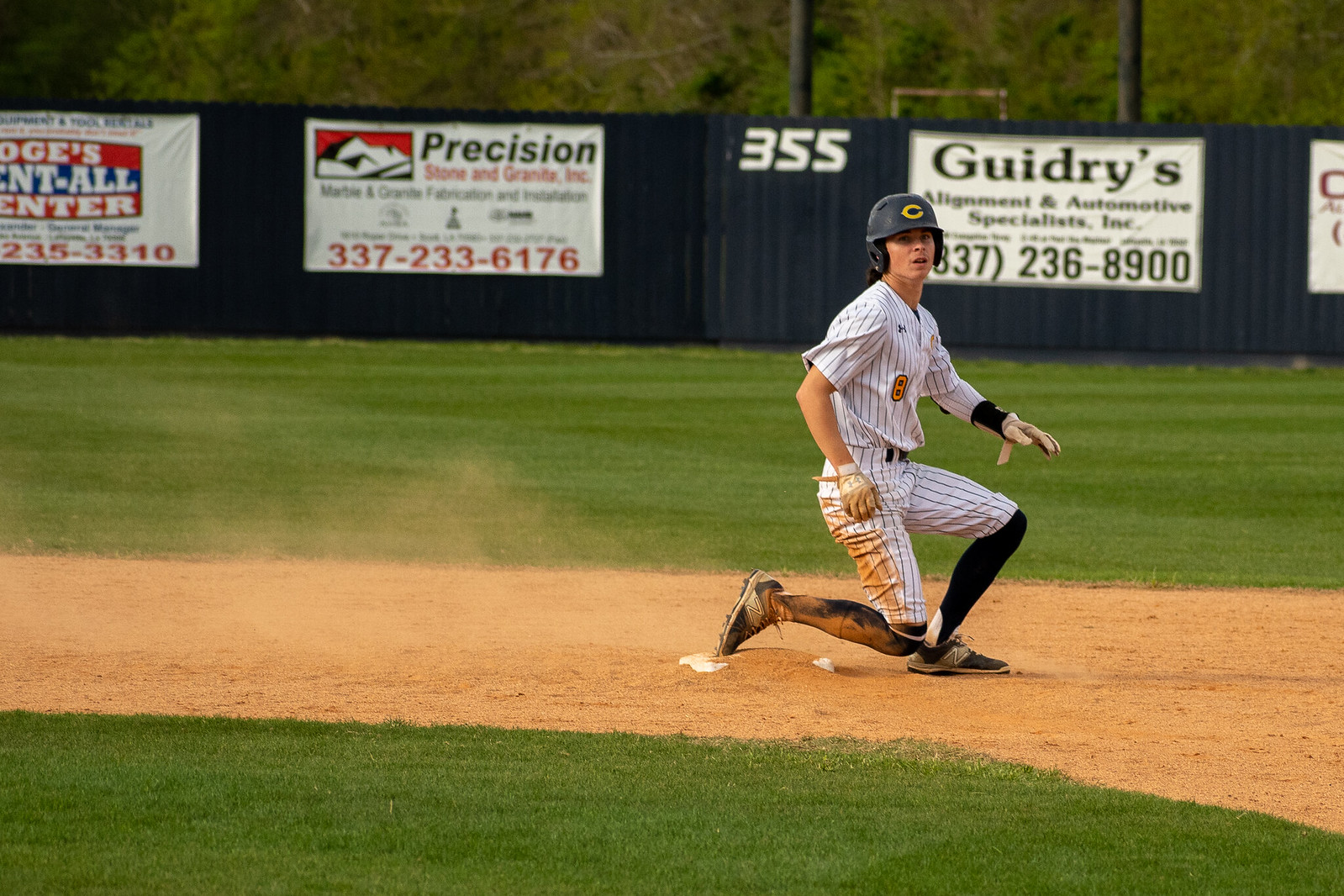The image captures a baseball player mid-game, kneeling on second base with dust swirling around his legs, indicating recent movement. Clad in a white uniform with black stripes and a helmet, he faces slightly toward the camera with his right side visible. His right knee is close to the ground, and his left leg is bent for support, while the tip of his right toes touches the base, which is a square padded cushion. The player, covered in sandy brown dirt, appears ready to run. Behind him stretches a well-manicured green field, leading to a blue wall adorned with advertisements. The prominent white banner reads "Precision Stone and Granite Incorporated Marble and Granite Fabrication and Installation," along with a red contact number "337-233-6176." Additionally, another advertisement displays "Guidry's Automotive Specialist." Tall, green-leafed trees and white poles rise beyond the wall, completing the backdrop of this dynamic sports scene.